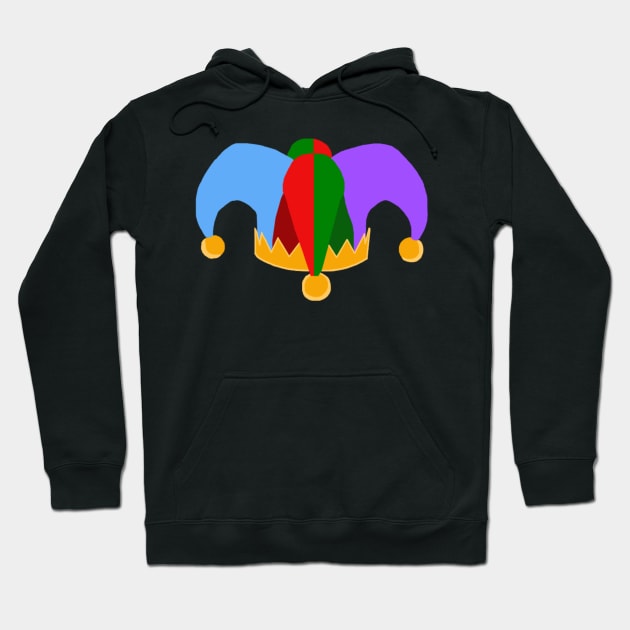This color photograph showcases a neatly pressed, black pullover hoodie displayed against a solid white, almost grayish backdrop. The hoodie features a hood with two laces for tightening, where the left lace bends slightly before straightening at the tip, and the right lace hangs straight. The hoodie also includes front pockets and has long sleeves that drape downward.

The central design element is a vibrant, multicolored jester's hat emblazoned on the chest. The jester's hat, complete with four "ears" or points, has a distinctive color scheme: the left ear is blue, the right ear is purple, and the middle sections are split into red and green. These colors mirror on both the front and back of the design. Each point of the jester's hat is adorned with a golden bell, and a crown is positioned at the base, adding to the regal and playful motif that captures one's eye.